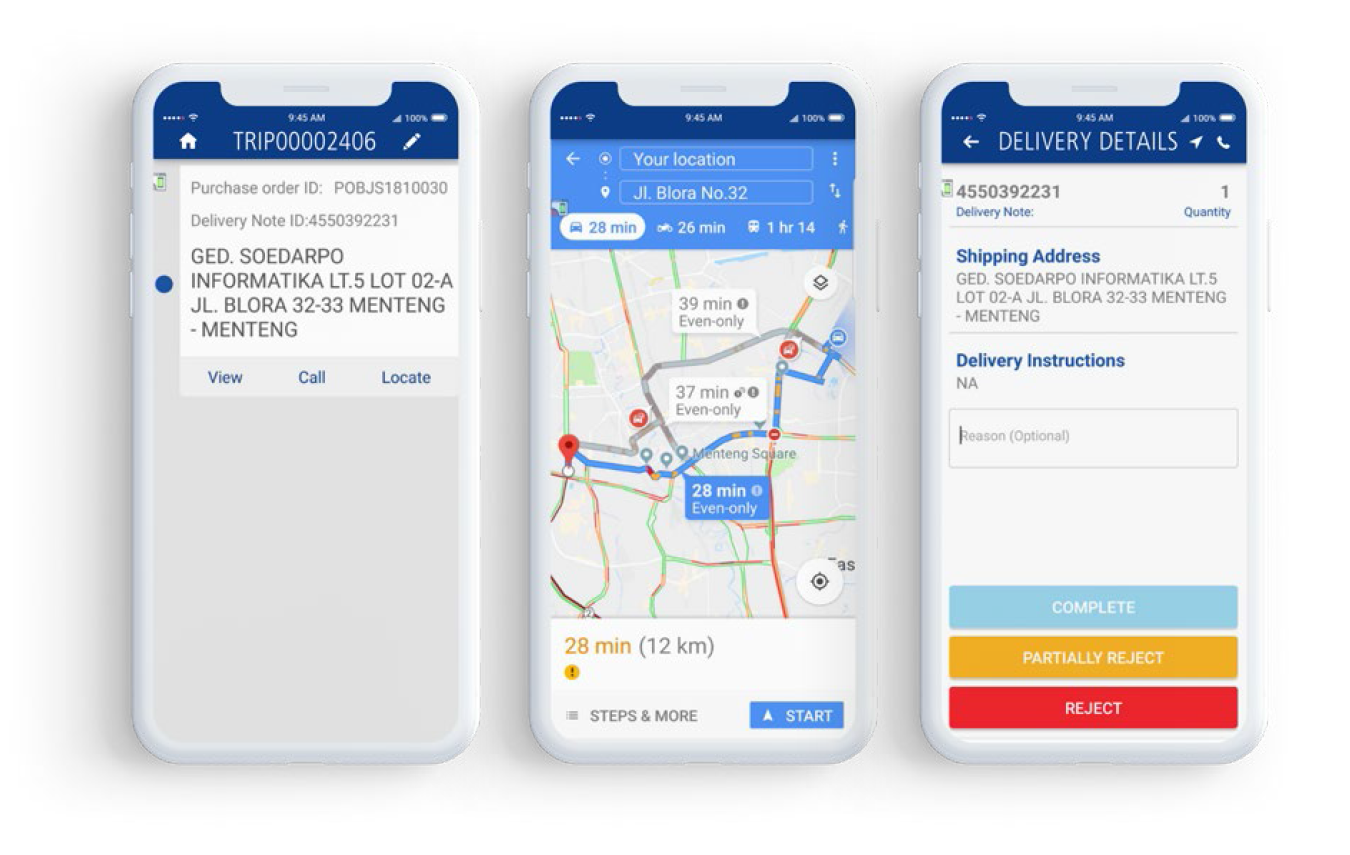The images consist of three consecutive screenshots of a mobile phone interface, which appears to be related to a delivery service, likely Uber Eats or a similar platform. The screen is predominantly white or light gray.

On each screenshot:
1. At the very top, there's a blue navigation bar featuring a home icon on the left, a title that reads “Trip 000002406” in white, and an edit icon on the right. Above this navigation bar, there is the standard notification bar for the phone.
2. Below the navigation bar, there is detailed trip information:
    - **Purchase Order ID:** P-O-B-J-S-1810030
    - **Delivery Note ID:** 4550392231
    - **Delivery Address:** GetSo Darpo Informatica LT.5 Lot O2A, JL Blora 32-33 Menteng
3. Further down, there are blue hyperlinks labeled "View," "Call," and "Locate." To the right of these hyperlinks, there's a small preview image of Google Maps displaying two marked points: "Your Location" and "JL Blora No. 32." It indicates a 28-minute drive or bike ride with an accompanying map icon, further detailed as 12 kilometers.
4. Below the map, there is an orange indication of travel time and distance (28 minutes, 12 kilometers), followed by a section titled "Steps and More."
5. The right part of the screen holds a prominent blue button with the label "Start."
   
Finally, at the bottom of the screen, there are delivery details such as shipping address, delivery instructions, and three action buttons:
- **Complete** (blue)
- **Partially Reject** (orange)
- **Reject** (red)

These elements combined form the interface for monitoring and managing active delivery trips, with explicit details for navigation, communication, and completion steps.